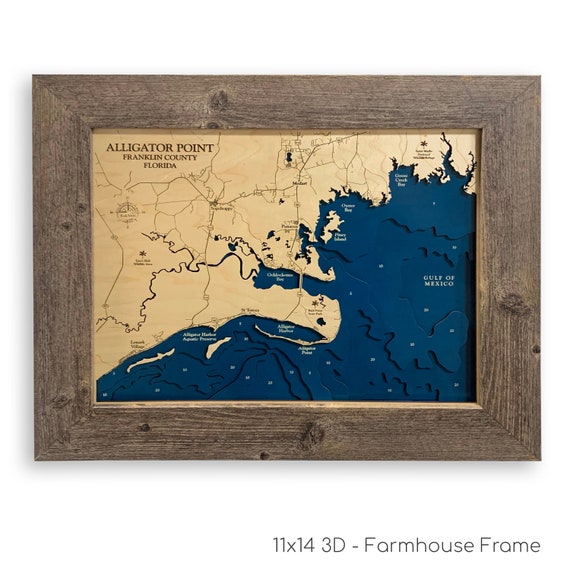This photograph captures a detailed map of Alligator Point, Franklin County, Florida, set within a distinctive 11x14 3D farmhouse frame. The frame is made of raw wood, featuring a natural, somewhat rugged appearance with visible knotholes, adding to its rustic charm. The map itself showcases the Gulf of Mexico in a vibrant blue, contrasting with the beige landmasses. Notable geographic features include peninsulas jutting into the water, labeled "Alligator Point," and several small islands. Black lines traverse the map, outlining different county sections and rivers. A round compass rose indicating the cardinal directions is also present, with south oriented at the bottom of the map. This framed map is displayed against a stark white wall, emphasizing its artisanal quality and the descriptive title beneath it, which reads "11 by 14 3D dash farmhouse frame."